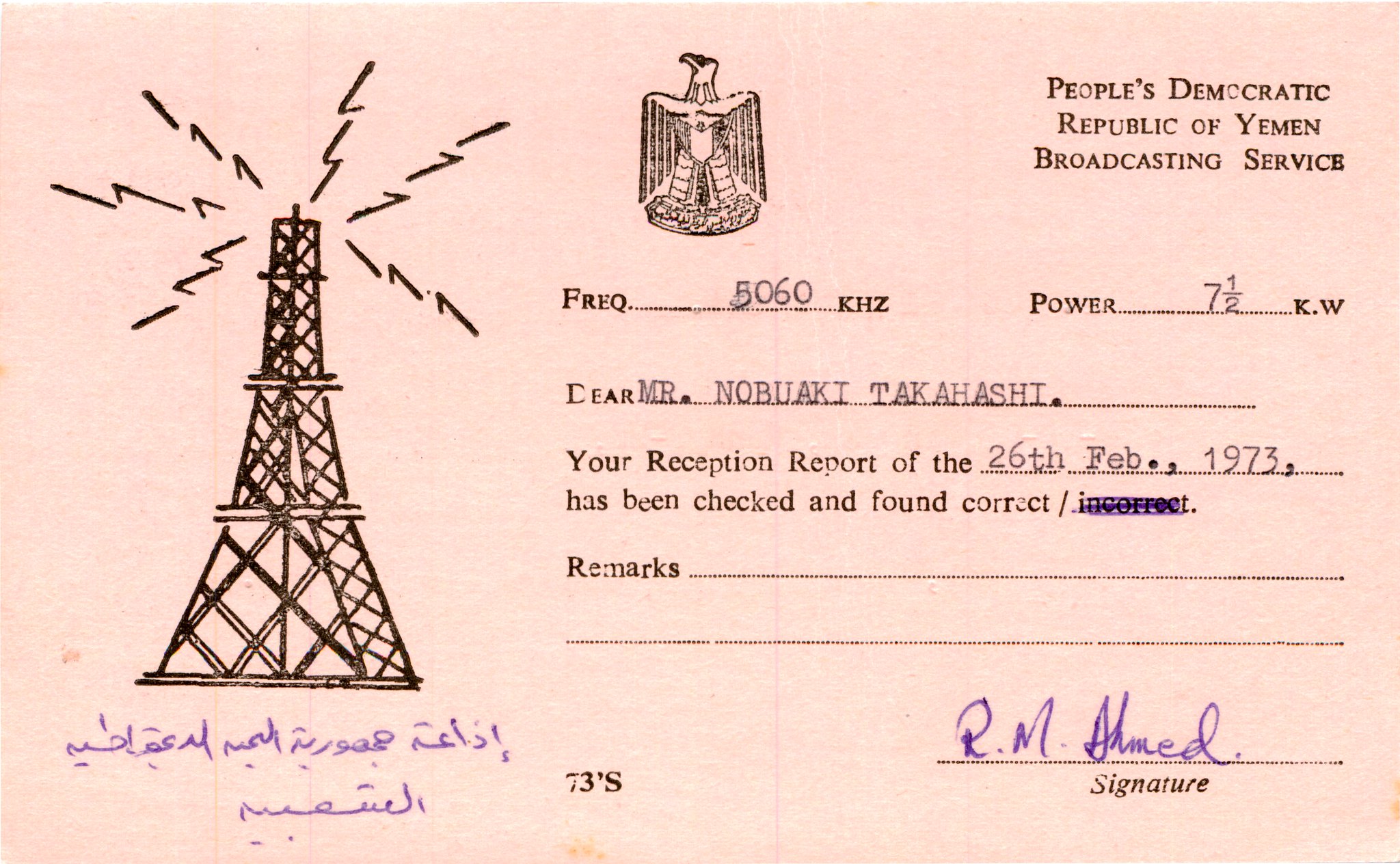The image depicts a peach or pink-colored reception report card issued by the People's Democratic Republic of Yemen Broadcasting Service in 1973. Centrally located on the card is an emblematic drawing of a phoenix, while the left-hand side features an illustration of a radio tower emitting broadcasting signals, represented by lightning bolt symbols. Underneath the tower, there's handwritten Arabic text. The card is addressed to Mr. Nobuaki Takahashi and confirms the accuracy of his reception report dated February 26, 1973. The report details include a frequency of 5060 kilohertz and a broadcasting power of 7.5 kilowatts. Notably, the card includes a section for additional remarks, which remains blank, and it is signed at the bottom by R. M. Ahmed in blue ink. The text and graphics are primarily in black.